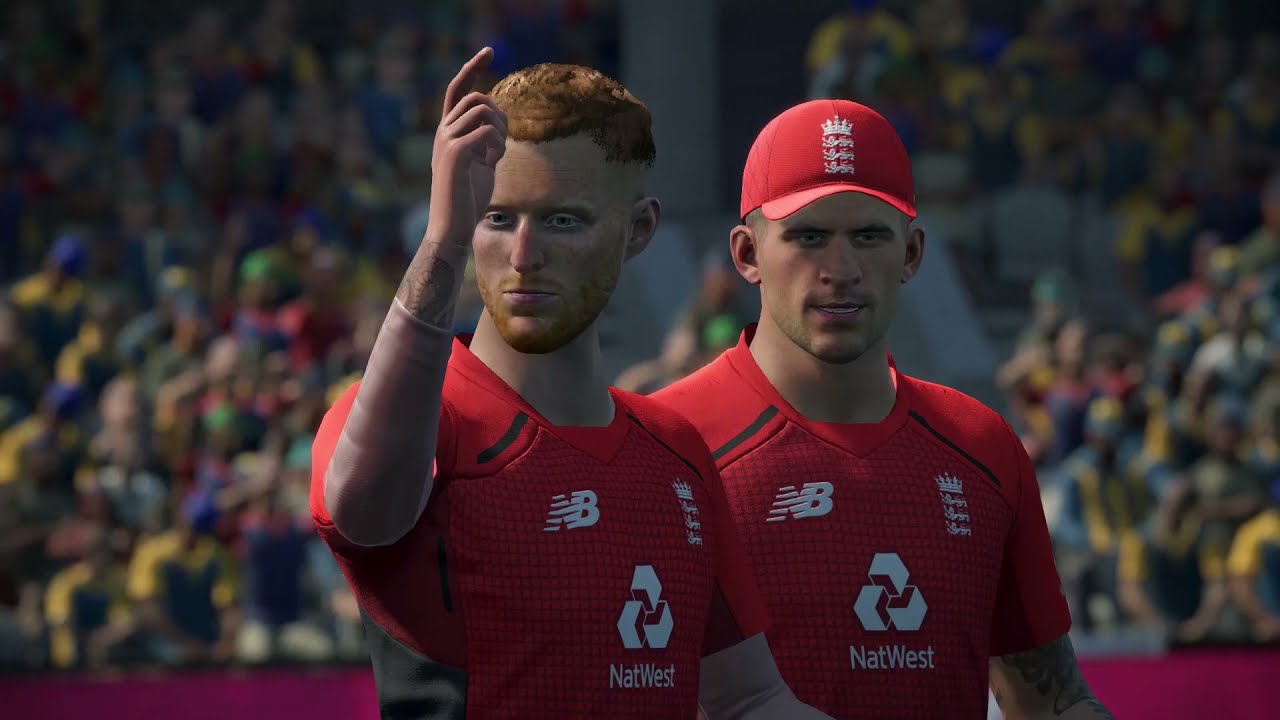The image is a detailed, computer-generated screenshot from a sports video game, featuring a stadium filled with a blurry crowd. Dominating the center are two digital athletes, clad in red short-sleeved jerseys emblazoned with sponsor logos including 'New Balance' on the pectoral and 'Nat West' with a logo of three intertwined squares on the center chest. Both athletes wear identical jerseys. The player on the left has short, cropped orange hair, an orange beard, and a forearm tattoo; he raises his right arm with a finger pointing skyward. Beside him is another player donning a red ball cap, marked with a foreign logo like the one on the jerseys. The vivid colors in the scene include shades of red, white, orange, tan, black, green, blue, and yellow, contributing to its cartoonistic, video-game style. Despite indications of various team sports, the exact sport remains ambiguous.